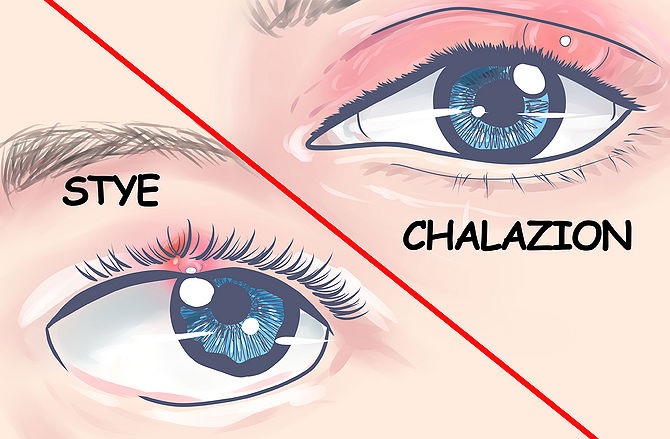This detailed poster showcases two illustrated human eyes within a rectangular frame with a 2:3 aspect ratio. A diagonal red line divides the image into two triangular sections. The top right section features a blue eye, presumably female, with black lettering that reads "Chalazion." This eye displays a round red sore situated above the eyelid. The lower left section also presents a blue eye with visible eyelashes and a part of the eyebrow, marked with a red inflamed area on the upper eyelid edge, labeled in black lettering as "Stye." The overall design incorporates hues of pink, blue, brown, and the striking red diagonal separator, making it suitable for a health-related website or ophthalmologist's reference material.